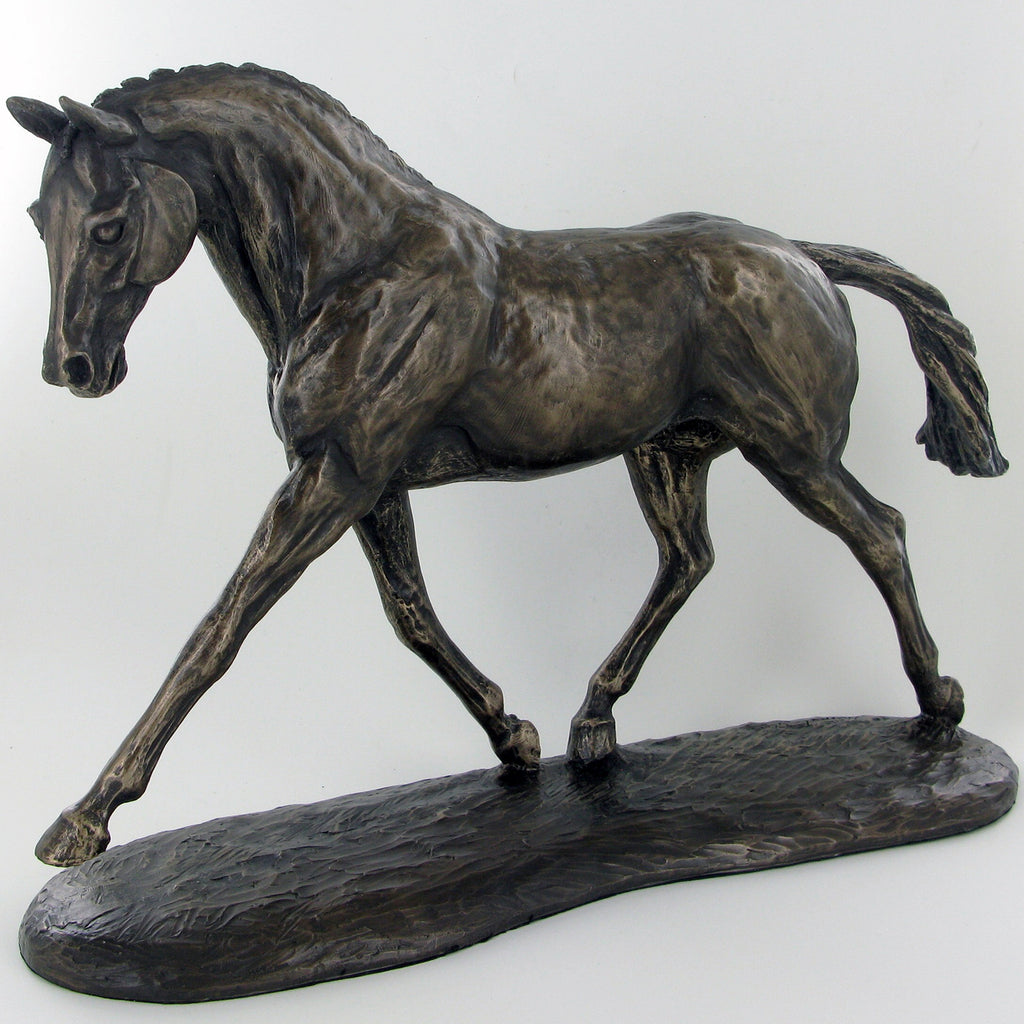This image captures a side-profile view of a detailed horse statue, which appears to be crafted from dark metal with hints of brown and gold. The horse, poised as if mid-walk, is centered on an elongated, horizontal base that mirrors its dark and metallic hues. The statue's three legs firmly rest on the base, while the fourth leg is raised, enhancing the sense of motion. The horse's head is positioned in the top left corner of the image, with its tail extending to the far right. Notably, the mane drapes down the side opposite the viewer, leaving the neck largely unobscured. The tail is trailing behind the horse, emphasizing its dynamic posture. The ears of the horse are perked, and one eye is visible, looking attentively to the left. Set against a whitish-gray background, the image focuses solely on the intricacies of the statue, highlighting its craftsmanship and lifelike detail.